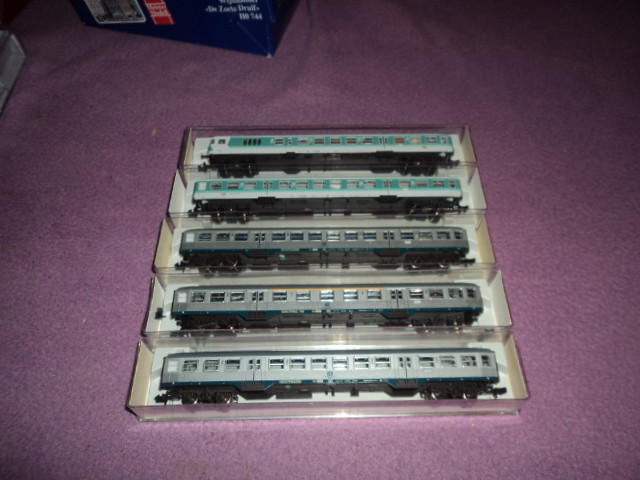The image showcases five model train cars, resembling passenger cars, all encased in clear display or retail boxes. They are neatly stacked, with three on the bottom and two on top, positioned on a purple burgundy colored rug. The bottom three cars are silver with blue trim near the wheels, while the top two are white with teal trim around the windows. The cars are aligned vertically but tipped slightly on their sides. Above the cars, a box with indistinct text is visible, and another box extends into the frame from the upper left corner. The purple carpet appears slightly rippled, indicating it might be a blanket. The overall scene is somewhat harshly lit. These model cars appear to be for preservation and display, appealing to collectors or enthusiasts.